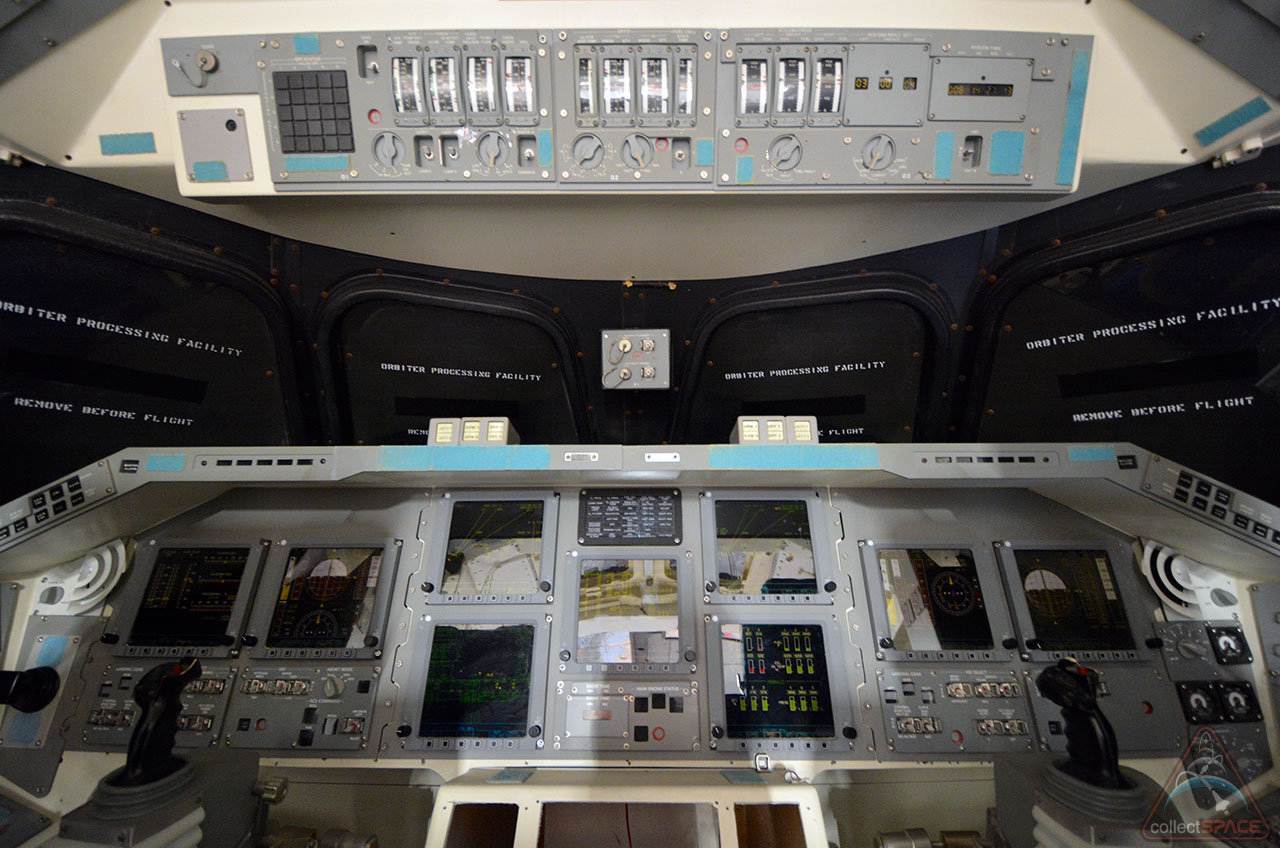This image showcases the interior of a space shuttle cockpit, distinguished by its detailed console featuring an array of switches, dials, and screens. Prominently, there are two large joysticks situated to the right and left sides, used for controlling the shuttle. The cockpit's color scheme comprises beige, black, and silver metallic elements, imparting a high-tech, utilitarian feel. The windows appear blacked out, bearing white text that reads "Orbiter Processing Facility Remove Before Flight," suggesting these panels are temporary coverings to be taken off prior to launch. Above the central console and along the top, additional monitors and control mechanisms are visible, emphasizing the complexity of the spacecraft's design. There's a central seat from which the pilot would operate the numerous controls, leaning back in a position typical for space launch. A watermark in the lower right corner reveals a logo and the text "Collect Space," identifying the image's source. The overall scene leaves viewers uncertain whether this is an operational cockpit or part of a training simulation, adding a layer of mystery to the setting.